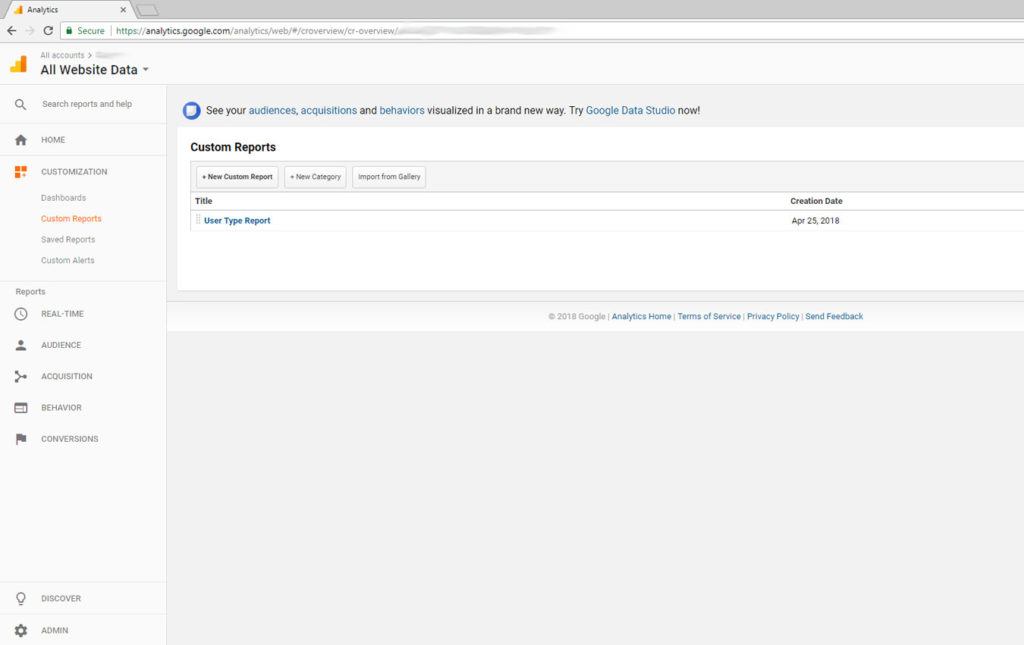In this screenshot, set against a predominantly white background with hints of gray, the interface of Google Analytics is displayed. The title "Website Analytics" is prominently written in the upper left corner of the window. The address bar at the top shows the URL: https://analytics.google.com. Below the URL, the first line in bold reads "All Accounts", followed by "All Website Data".

There is a vibrant graph in shades of orange and yellow visible on the page. 

The left side of the image features a vertical navigation menu containing the following items, listed from top to bottom: 
- Search Reports and Help
- Home
- Customization
  - Dashboards
  - Custom Reports
  - Saved Reports
  - Custom Alerts

A faint gray line separates this section from another list below:
- Reports
  - Real-Time
  - Audience
  - Acquisition
  - Behavior
  - Conversions

On the main page, the text "See your audience's acquisitions and behaviors visualized in a brand new way. Try Google Data Studio Now" is prominently displayed. Below this message is a custom report titled "User Type Report" with the creation date specified as April 25th, 2018.